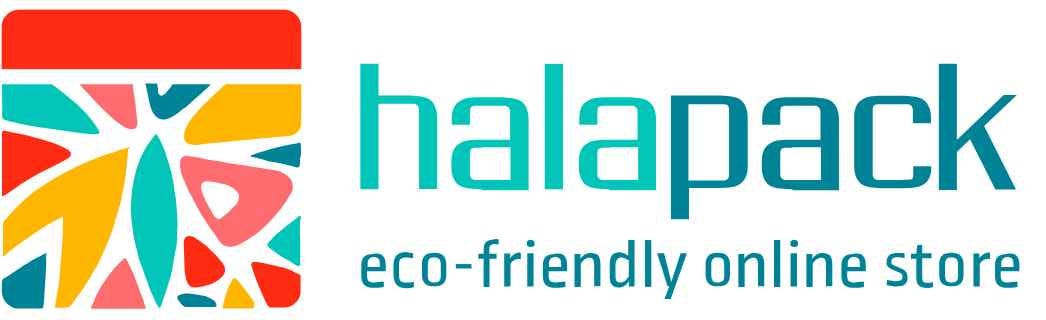The image is a company logo designed to look like a label. It features a sleek, contemporary, and almost robotic-like font, with the text "HALA Pack" split equally in color—"HALA" in turquoise blue and "Pack" in a darker teal blue. Below this, in teal blue, the wording "Eco-Friendly Online Store" is positioned. To the left of the company name and tagline, there is a colorful icon that resembles a jar with a red screw-on lid, set atop a white rounded square. This icon contains various geometric shapes in yellow, peach, blue, and salmon colors, giving it a vibrant and multi-colored appearance. The entire design sits against a white background.